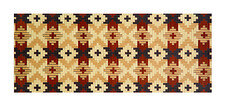The image depicts a small horizontal rectangle that appears to be a fabric with a geometric, quilt-like pattern. The intricate design features vertical stripes and diamond shapes in a harmonious blend of light yellow, orange, dark red, and black. The pattern is meticulously detailed: it showcases tiny black and red crosses within diamond shapes, creating a series of larger vertical stripes.

Prominent within the pattern are seven narrow columns, each capped by a large black X at both the top and bottom. Interspersed between these columns are six additional ones, each featuring diagonal squares and plus signs. The central areas of these columns exhibit darker gold diamonds centered by red crosses, set against a backdrop dominated by red with small blue crosses and yellow diamonds. Adding complexity to the design, certain columns display an eight-pointed star, partially rendered in dark colors and partially in red. The overall aesthetic of the fabric is vibrant yet orderly, characterized by its balanced use of color and geometric forms.